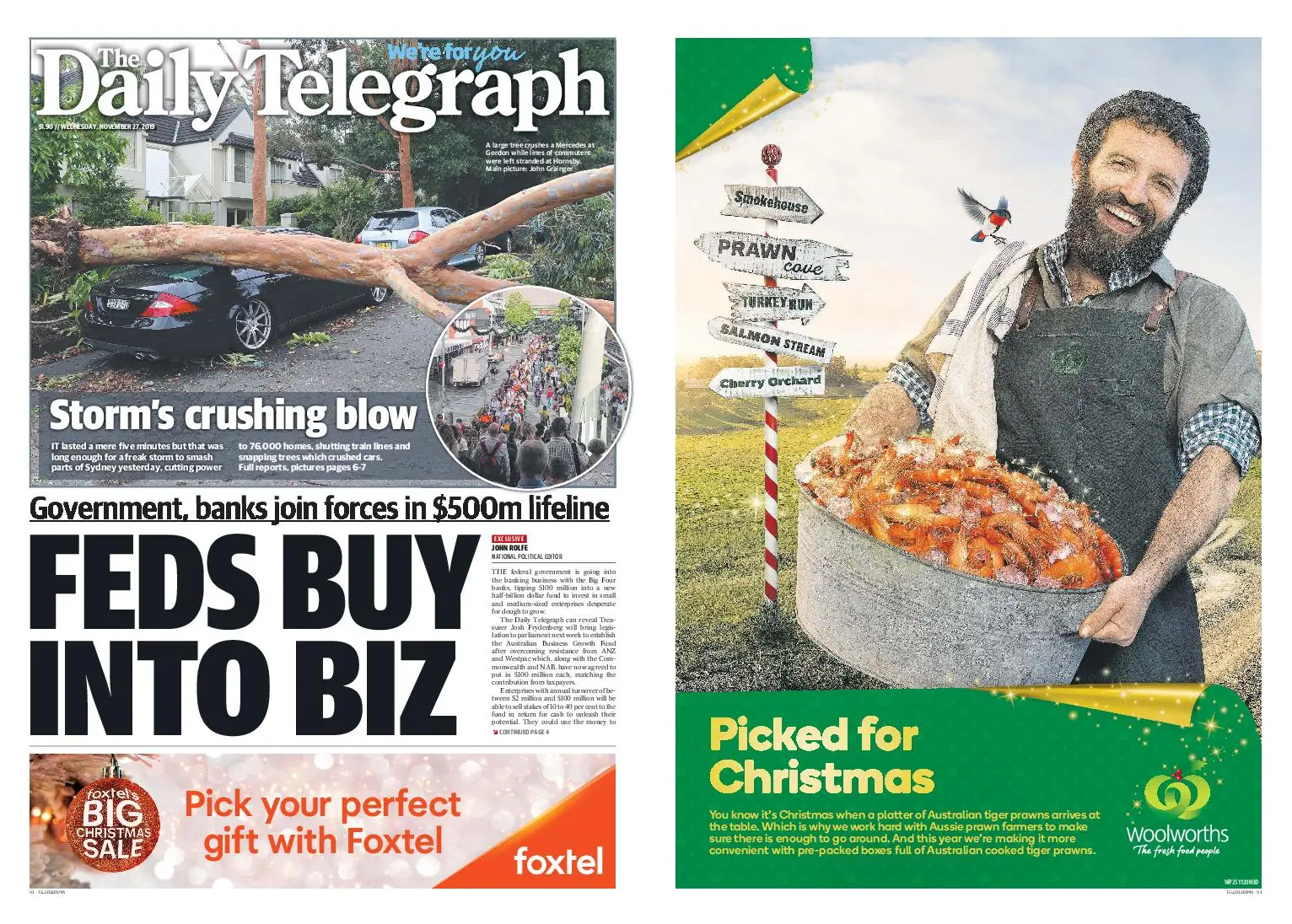The image showcases two pages from a magazine. On the left page, "The Daily Telegraph" is prominently displayed at the top. The page features a photograph of a street lined with two parked cars, one gray and one black. The black car has been significantly damaged by a fallen tree. Above this image, a headline reads "Storm Crushing Blow," followed by subtext mentioning "Government, banks, joint forces, $500 million lifeline fed by an abyss." This page is filled with several paragraphs of text, though they are too small to read. At the bottom, an advertisement for a "Big Christmas Sale" with the tagline "Pick your perfect gift with Foxtel" is visible.

The right page presents an image of a road sign with five different direction markers against a green background. The road sign stands atop a red and white striped pole. Accompanying text in gold reads "Pick for Christmas." Below this, an unreadable block of text is present, alongside the recognizable Woolworths logo.